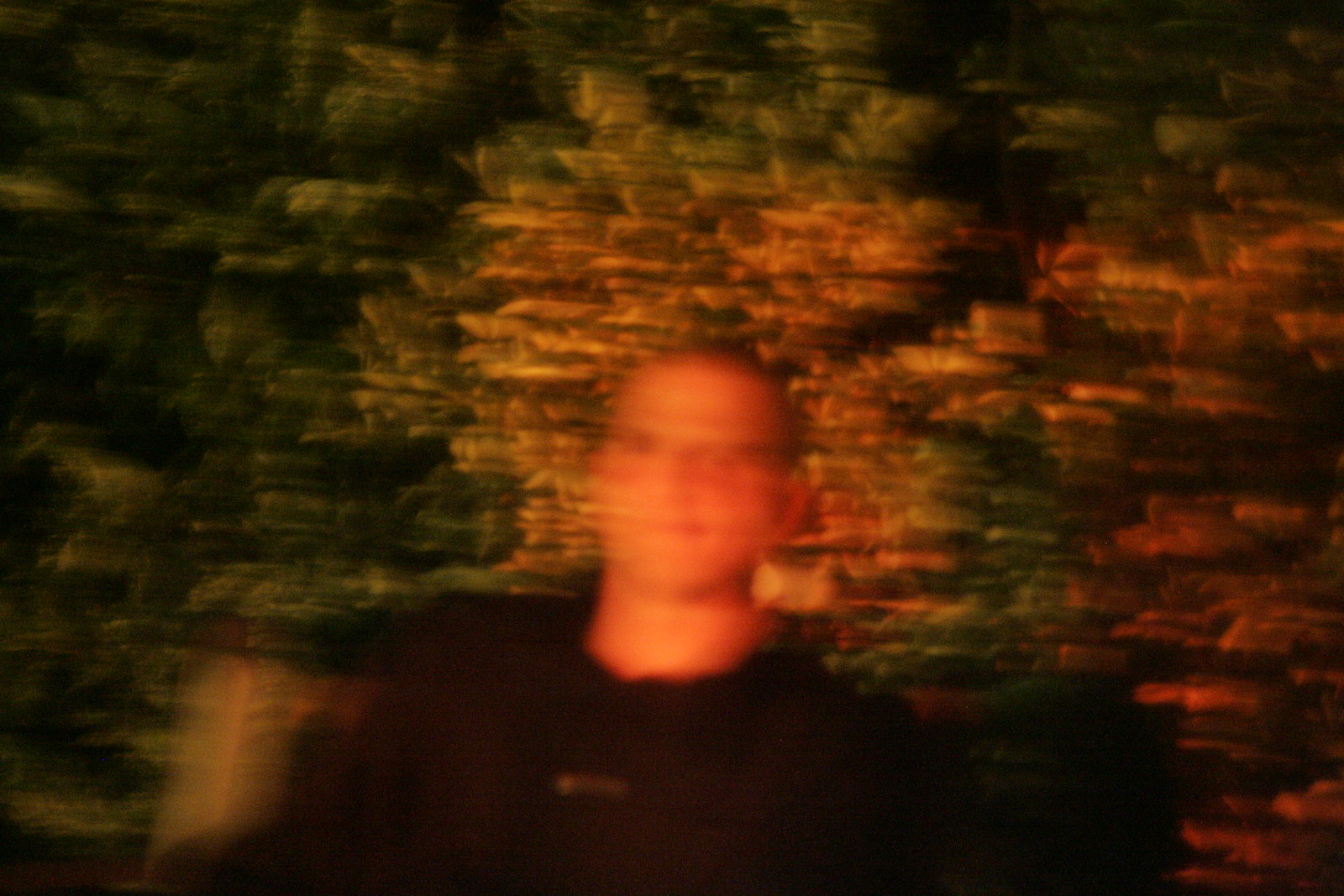A man with a shaved head is pictured from the chest up, sitting and smiling at the camera. He is wearing a black sweater over a black shirt, which has an indistinct label on it. The image is noticeably blurred, making the finer details of his face hard to discern, though his smile is still visible. Behind him to the left, there's a hint of a chair or bench. The backdrop consists of dense vegetation, featuring green and yellow hues, suggesting a large bush. The overall scene is dimly lit, indicating it might have been taken during nighttime, with darker areas present on both the left and right sides of the photo.